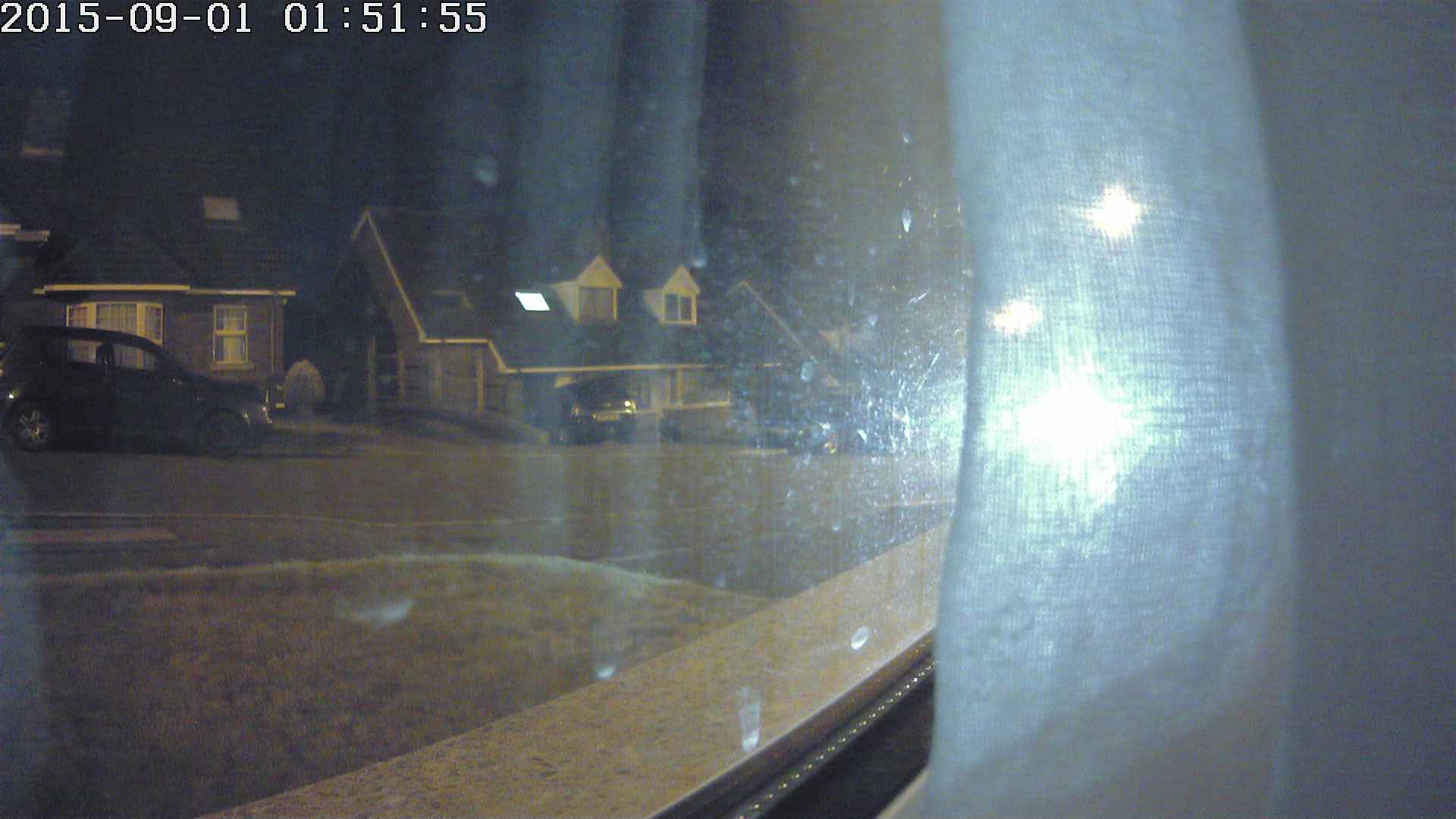Captured at 01:51:55 on September 1, 2015, this nighttime scene presents a detailed vista through a bedroom window adorned with light blue curtains. Opposite the window, two brick houses stand on a quiet street. The first house has a black car parked in front, while the second house, with an upstairs light turned on, features a car both in the driveway and parked out front. The street is illuminated by two streetlights, and distant car lights are visible approaching. The ambiance of the night is subtly shadowed but provides a clear view of the serene neighborhood.